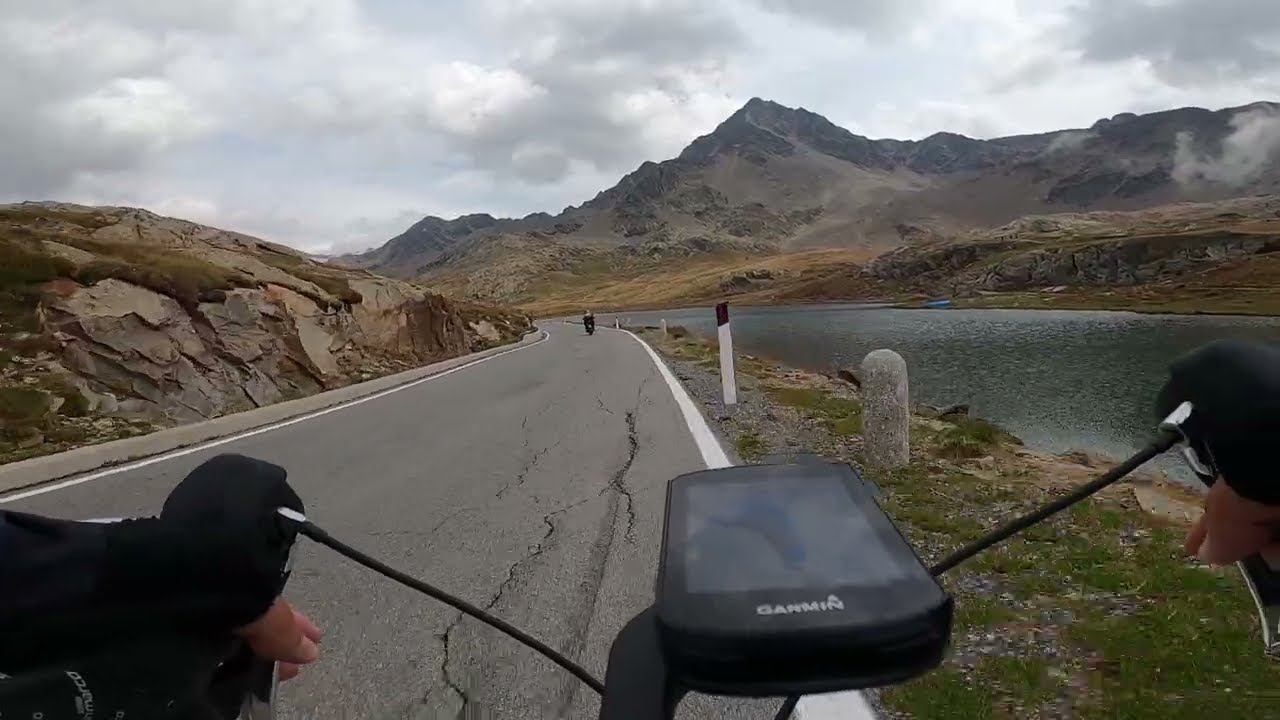In this detailed image, we see a single-lane asphalt road positioned directly in the center, suggesting a first-person view from a motorcyclist riding through a mountainous area during the day. The road is gray and cracked, with white lines painted on either side. Central to the foreground is a motorcycle's handlebars, with the rider's gloved hands visible and a Garmin GPS device mounted on the front.

On the right side of the road, there is a quiet river, about 10 to 20 feet from the edge, with beams positioned as barriers to prevent vehicles from veering into the water. The grassy and rocky terrain accompanies the riverbank. To the left, there's a rocky hill or granite mountainscape dotted with patches of green moss and foliage. 

In the background, a larger mountain range extends across the horizon beneath a sky that is partly cloudy, with gray clouds hinting at the possibility of an impending storm. The overall color palette includes shades of white, gray, brown, tan, black, and green. Another motorcyclist can be seen further down the road in the distance, adding depth to this scenic and adventurous landscape photograph.